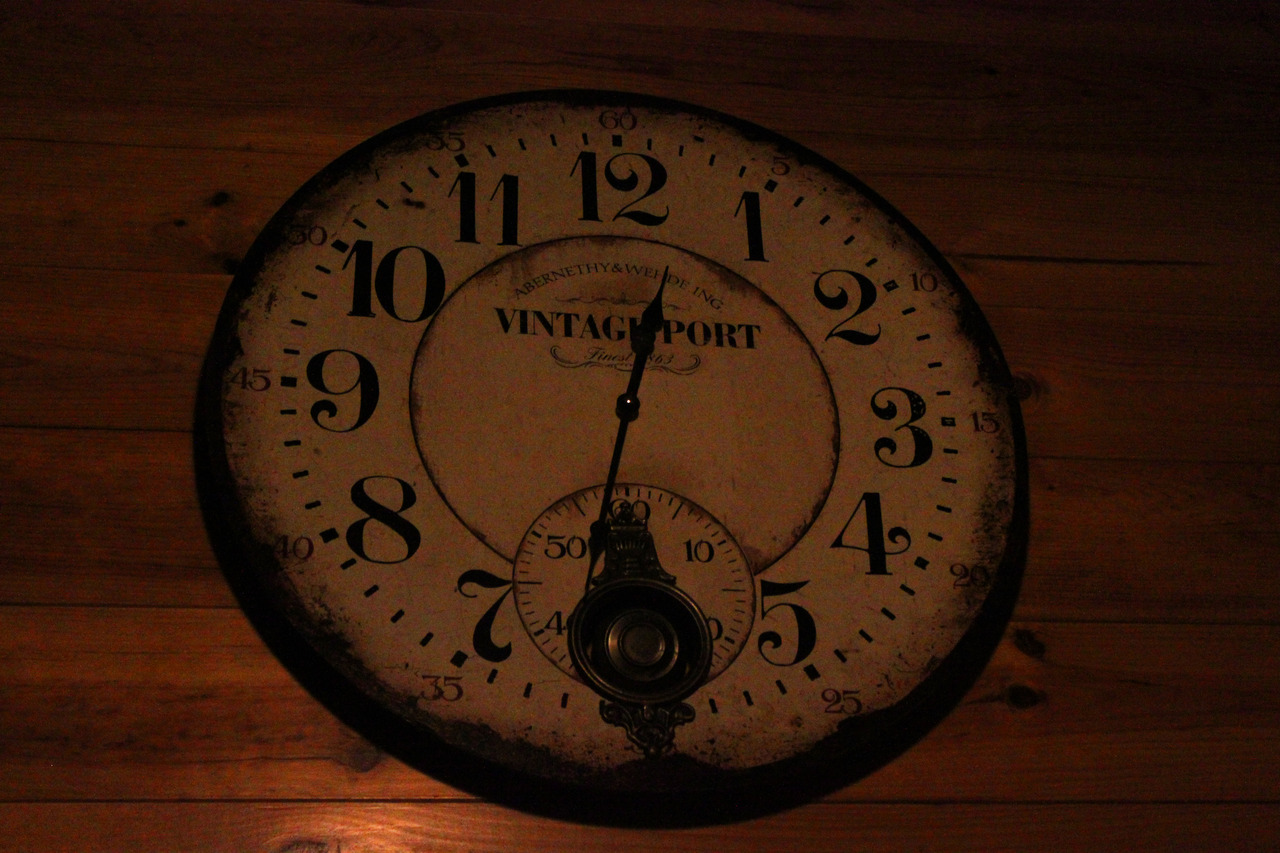This underexposed, dark photograph reveals an antique wall clock with significant rust framing its edges, positioned against a backdrop of dark wood with visible knots, likely pine. The clock face, yellowed to an almost brown hue, displays large, old-fashioned numerals from 1 to 12, with minute markers at every five-minute interval, clearly labeled. The main hour-hand shows the time as approximately 12:32, and partially obscures text that reads "Vintage Port," possibly celebrating a type of wine. There is additional, hard-to-decipher cursive lettering above and below this main label, potentially indicating "Abernathy and Wending." The clock also features a smaller sub-dial where the number 6 usually resides, marked with the numbers 10, 40, and 50, suggesting an additional timekeeping function, such as a stopwatch or second-hand. In the lower section of the clock face, a metallic, round object resembling a pendulum or a decorative fixture, possibly depicting a Liberty Bell, adds to its antique character.